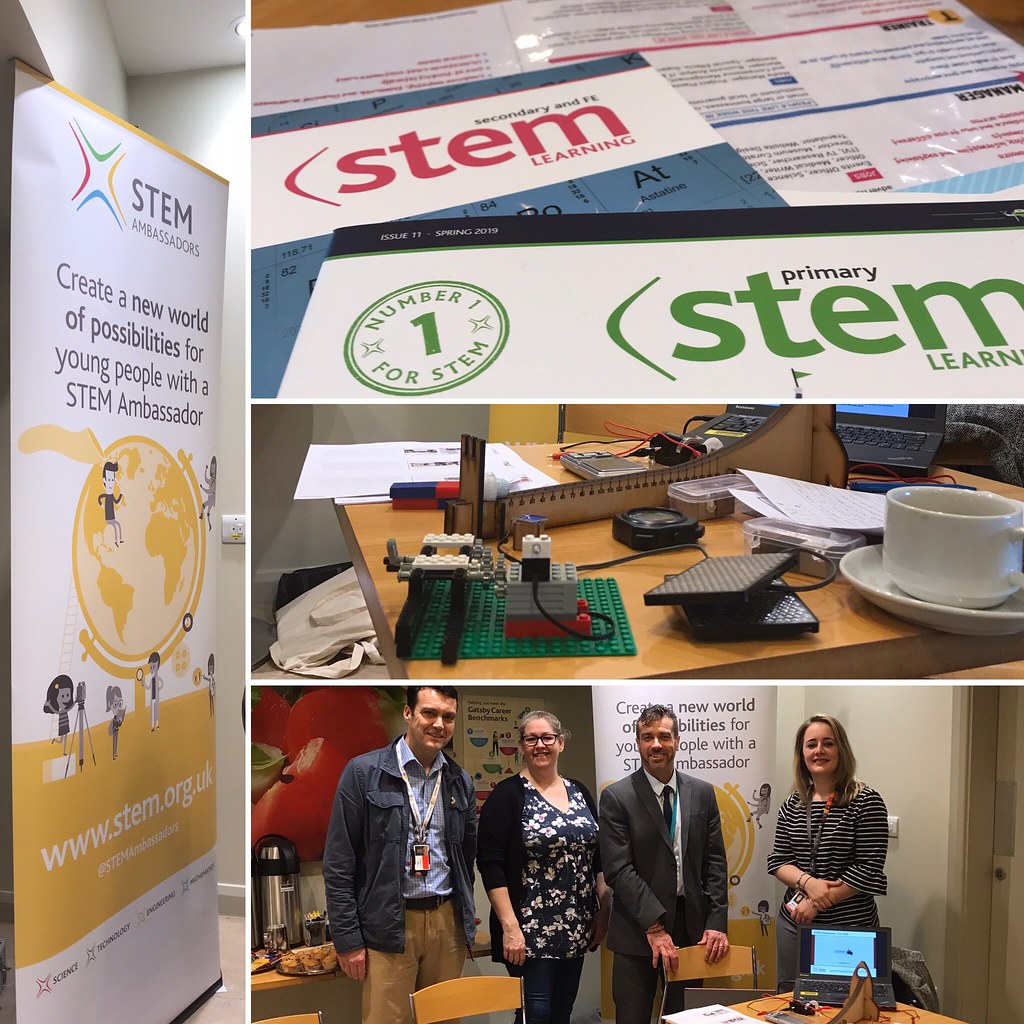This is a detailed multi-panel collage image with a square orientation, prominently featuring themes of STEM (Science, Technology, Engineering, and Mathematics) education and outreach. The vertical panel on the left depicts a promotional poster for STEM Ambassadors. This poster showcases colorful intersecting lines of red, green, yellow, and blue beside the word "STEM", and highlights the slogan, "Create a new world of possibilities for young people with a STEM Ambassador." Below the slogan, there's an illustration of a globe in gold, surrounded by children engaged in various scientific experiments, such as one with a tripod and others examining objects with magnifying glasses. The URL "www.stem.org.uk" is prominently displayed in white text on a gold background.

On the right side, three horizontal panels are stacked on top of each other. The top panel features an array of STEM literature, including brochures and flyers labeled "STEM Learning." The middle panel provides a close-up view of a desktop setup, which includes a laptop, a white coffee cup on a saucer, and some Lego-based gadgets resembling a simple motorized contraption. The backdrop consists of educational scales and tools. The bottom panel shows four adults—two men and two women—standing in front of a table and looking directly at the camera, smiling. They wear placards around their necks and are surrounded by posters promoting STEM activities, suggesting a meeting or demonstration related to STEM initiatives. This collage combines elements of graphic design, illustration, and photographic realism to convey a vibrant and dynamic STEM educational environment.